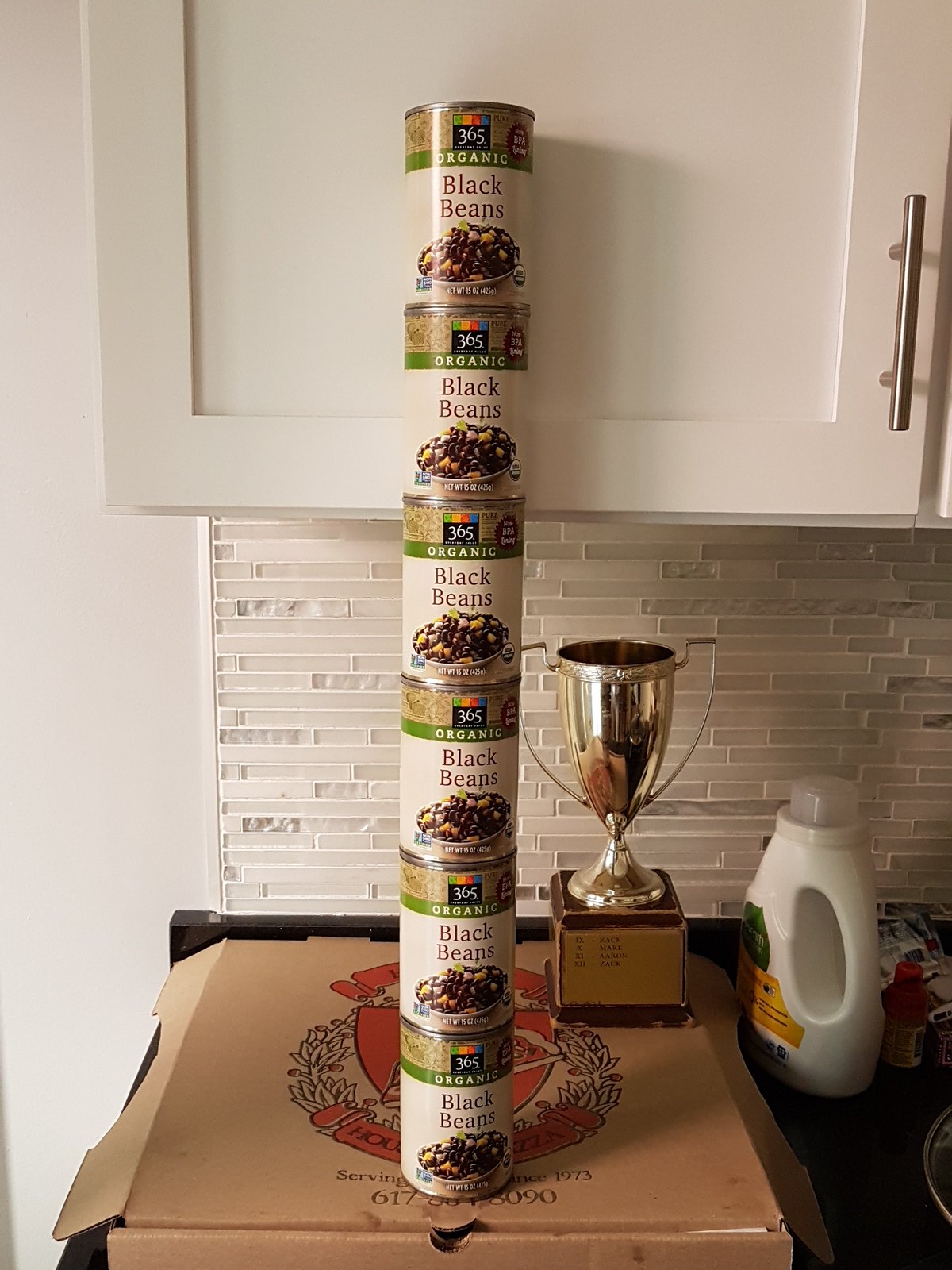In this detailed photograph taken in a kitchen, six cans of 365 Organic Black Beans are meticulously stacked on top of each other, forming a vertical tower atop a pizza box. Each can displays a consistent label: a brown top featuring a green banner that reads "organic," transitioning to a white background with "black beans" written in black text, and adorned with an image of a bowl of black beans. The colorful 365 brand logo, with its bars of green, orange, red, and blue, crowns each label.

The scene unfolds on a black countertop, barely visible beneath the pizza box, which itself sports a large, red central logo. To the right of the cans, there is a white bottle resembling a laundry detergent container, complete with a plastic top. Additionally, a golden trophy with a distinct cubed base is placed near the cans atop the pizza box.

The background is set against a kitchen backsplash consisting of thin, elongated tiles resembling a brick pattern, set beneath white cabinets with silver handles. The cabinets, coupled with a plain white wall on the left, frame the main subject of the photo, emphasizing the neatly arranged cans and their surroundings.